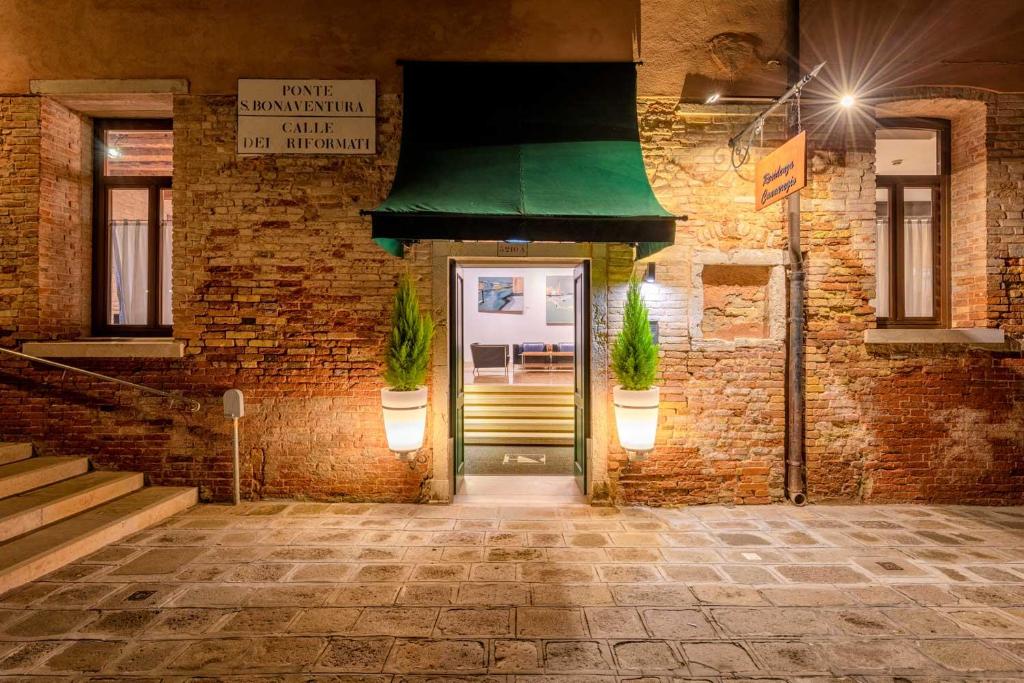The image captures a rustic, old-school village scene taken in the evening. The focal point is a quaint brick and stone building with a central entrance featuring green double doors that open inward, revealing a brightly lit interior. This entrance is marked by a green awning above, which is flanked by two illuminated potted plants that also serve as lights. These pots house small green pine-like trees. The building's façade includes rectangular windows on either side of the awning. 

In front of the building lies a stone pathway composed of brown pavers bordered with white, resembling driveway stones. A set of five or six steps leads up from this pathway to the entrance, where the interior shows paintings on a white wall and lounge chairs beneath them. To the left of the building's entrance, there is another staircase ascending, while in the upper left corner, a sign reads, "Ponta S Bonaventura Cali De Reformati," suggesting an Italian or Spanish influence. An additional sign hangs at an angle to the right of the awning, though its text is not clearly visible. A large spotlight can also be seen in the upper right corner of the image, illuminating the scene.